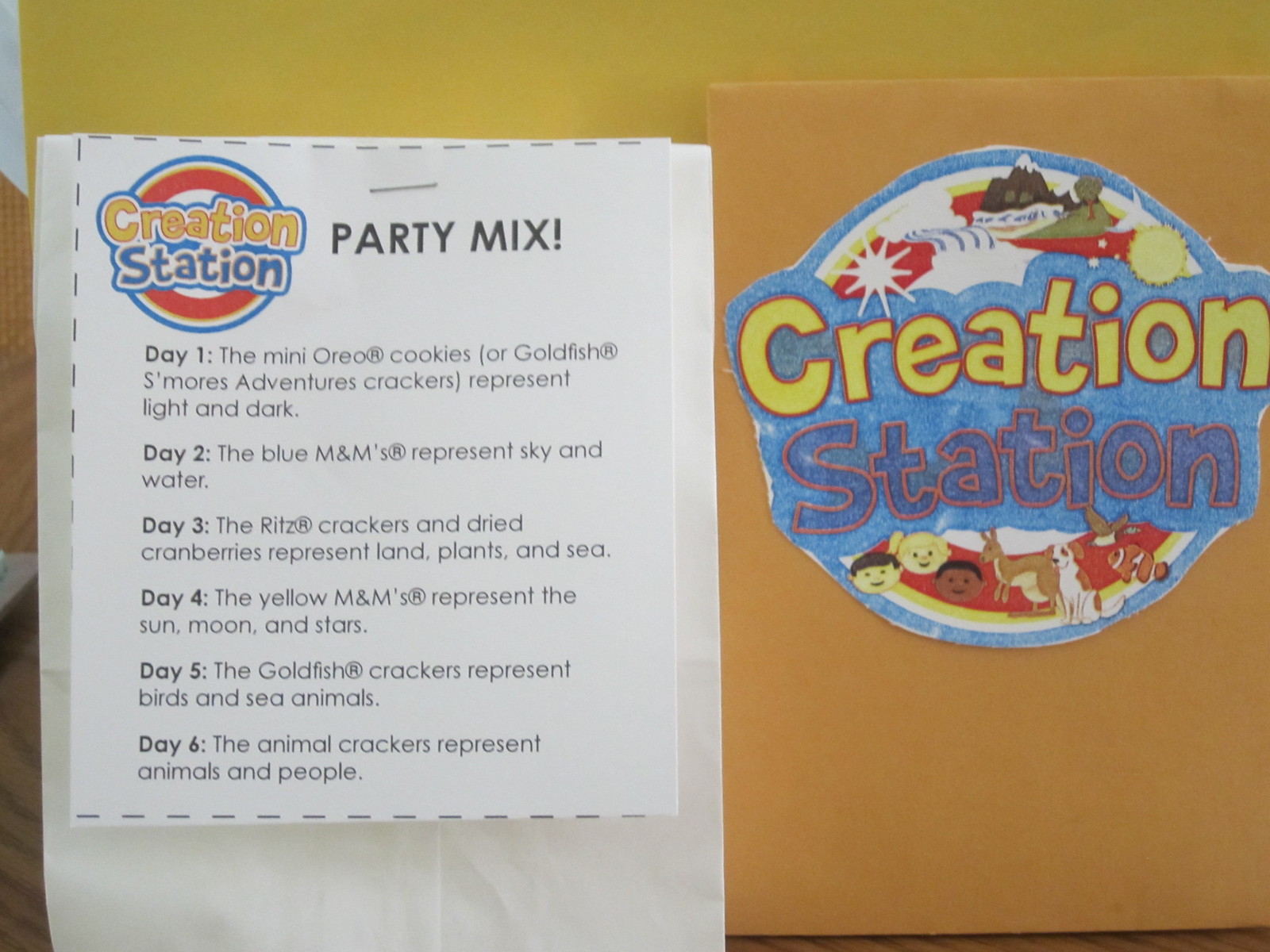The image showcases a vibrant and educational Creation Station Party Mix, accompanied by detailed descriptions for each day. On the left side, a white piece of paper features a colorful Creation Station logo in yellow and pink, set against red, green, and blue circles, along with the title "Party Mix!" in bold. This white paper details a seven-day creation-themed snack journey: 

- **Day 1:** Mini Oreo Cookies or Goldfish S'mores Adventure Crackers represent light and dark.
- **Day 2:** Blue M&Ms symbolize the sky and water.
- **Day 3:** Ritz Crackers and dried cranberries stand for land, plants, and sea.
- **Day 4:** Yellow M&Ms signify the sun, moon, and stars.
- **Day 5:** Goldfish Crackers embody birds and sea animals.
- **Day 6:** Animal Crackers depict animals and people.

On the right side, a green paper features the Creation Station logo again, emphasizing the theme. The playful logo includes little kids and animals, colored in red, yellow, and blue. The overall background of the image is a cheerful yellow. This setup illustrates how to create a fun and meaningful trail mix or party mix using everyday snacks like Ritz Crackers, M&Ms, various cookies, and dried berries, with each element representing different parts of a creation narrative.